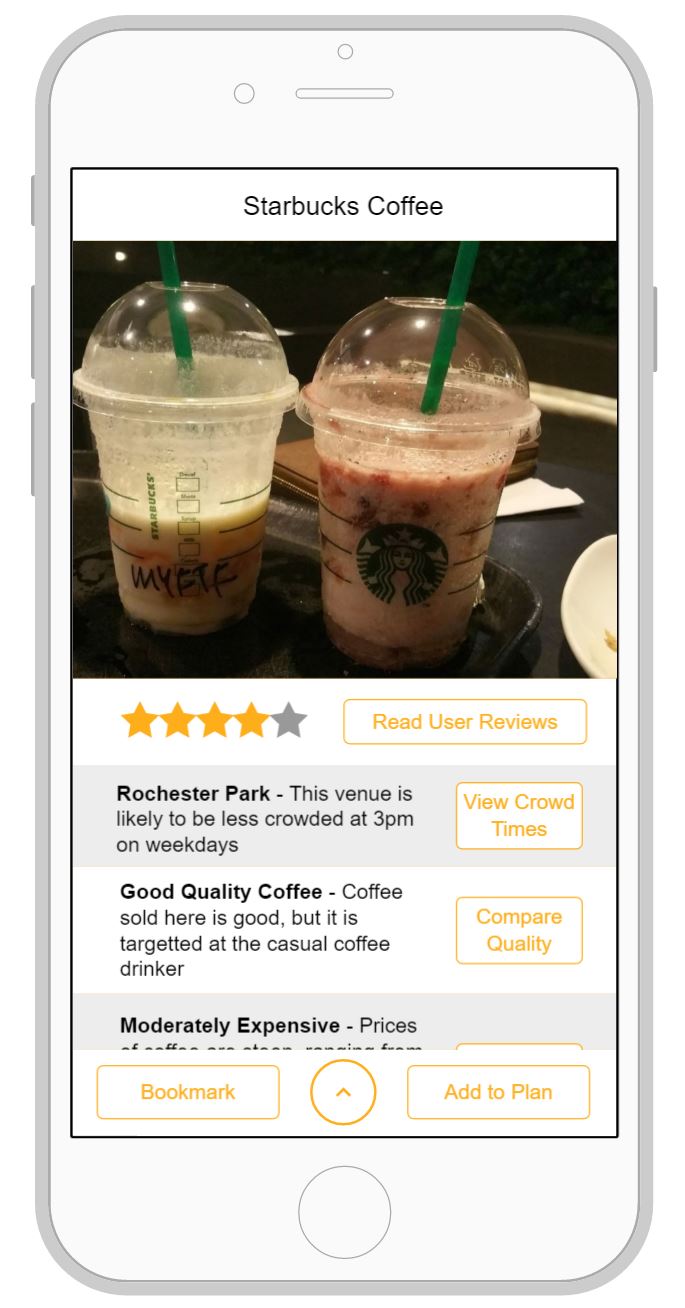The image is a digitally crafted screenshot designed to look like it is displayed on a silver-bordered smartphone. This virtual phone features three buttons on the left side and one on the right side. Within the phone screen, the actual screenshot showcases a review of Starbucks Coffee. 

At the top, the screenshot has a black bar with the text "Starbucks Coffee" prominently displayed against a white background. Below this header, there is a photograph of two partially consumed cold Starbucks beverages, each with a green straw. The left drink has a label "M-Y-F-T-F" visible, while the right drink's label is obscured, showing only the Starbucks logo. 

Underneath the photo, there is a rating section that displays "four stars out of five." An orange button labeled "Read User Reviews" follows. 

The subsequent row, backed by a gray background, starts with bold text that reads "Rochester Park." A note follows, indicating that this venue is likely to be less crowded at 3 p.m. on weekdays. Another orange button labeled "View Crowd Times" is placed here.

The next section boasts the phrase "Good Quality Coffee," followed by the comment, "Coffee sold here is good, but it is targeted at the casual coffee drinker." A clear, orange button labeled "Compare Quality" is also included in this row.

Continuing in gray, the following row comments on the pricing, stating "Moderately Expensive." 

At the bottom of the screenshot are two buttons: the left one says "Bookmark" and the right one says "Add to Plan."